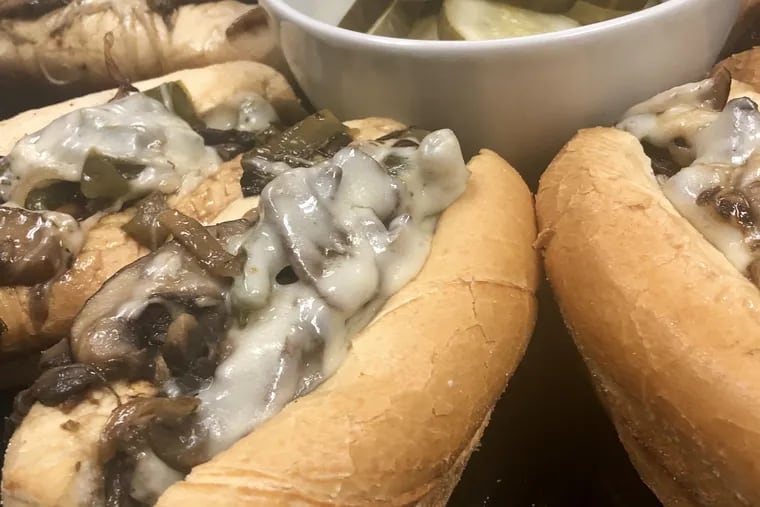The image shows a close-up view of an appetizing platter of Philly cheesesteak sandwiches arranged in an eye-catching manner. A pristine white ceramic bowl, filled with pickles, sits at the center of the platter, acting as the hub around which four heavily-stuffed Philly cheesesteak sandwiches are positioned like spokes of a wheel. Each sandwich is packed with grilled onions, peppers, and a generous amount of melted cheese, making them look irresistibly delicious. You can also spot various types of mushrooms smothered in cheese, further adding to the hearty appeal. The soft, well-browned buns are accompanied by an inviting white gravy-like sauce. The overall presentation is mouth-watering, as the combination of ingredients and the detailed arrangement suggest a meal ready to be enjoyed.